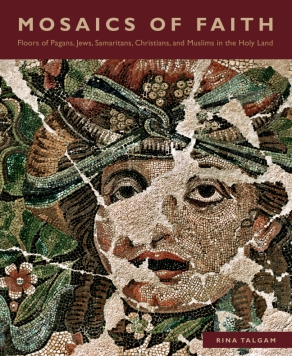The book cover titled "Mosaics of Faith" features a maroon background at the top with the title and subtitle written in beige, all-caps font. The subtitle reads, "Floors of Pagans, Jews, Samaritans, Christians, and Muslims in the Holy Land." Below the text is an aged but colorful mosaic depicting a woman's face, adorned with green tiles and reddish brown tiles, and a partially damaged surface that reveals white areas, akin to corrosion or wear. The woman appears to have a green ribbon tied around her forehead, with some features like her nose and mouth showing signs of damage, which gives a fragmented look to the mosaic. Surrounding the face are different abstract shapes and plant-like figures. In the lower right-hand corner of the cover, the author's name, Nina Talga, is clearly printed.